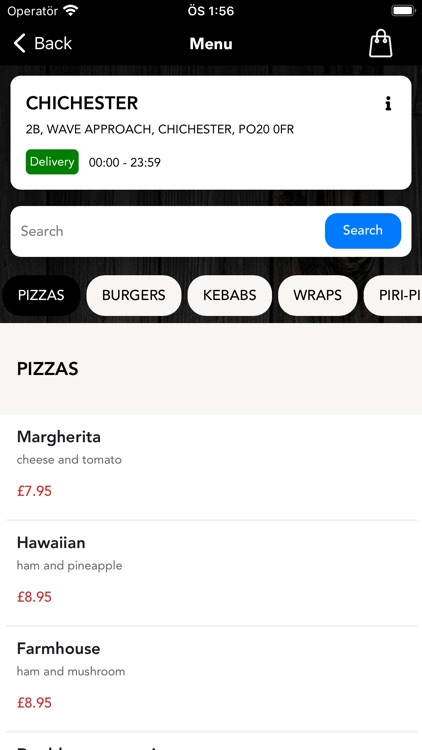The image is a screen capture of a smartphone displaying a food ordering application. The operating system and current time are indicated at the top, showing 1:56. The battery icon appears fully charged, and the Wi-Fi signal is strong. The top menu bar includes an icon resembling a small bag. The overall background of the screen is black, while the central area is white.

In the middle of the screen, there is an address that reads "Chickister 2B Wave Approach, Chickister P020 OFR," suggesting a location in Britain. Beneath this, the delivery time frame is indicated as "0 to 23:59." A search bar is located near the top, allowing users to search for items.

Below the search bar, there are several clickable categories for food items. The first category, "Pizzas," is highlighted without a button around it, whereas other categories such as "Burgers," "Kebabs," "Wraps," and a partially visible "Peri-" category have white buttons with black lettering.

The selected category is "Pizzas," displaying the following options and prices:
- Margherita (Cheese and Tomato) for £7.95
- Hawaiian (Ham and Pineapple) for £8.95
- Farmhouse (Ham and Mushroom) for £8.50

The user appears to be awaiting delivery of their selected items.